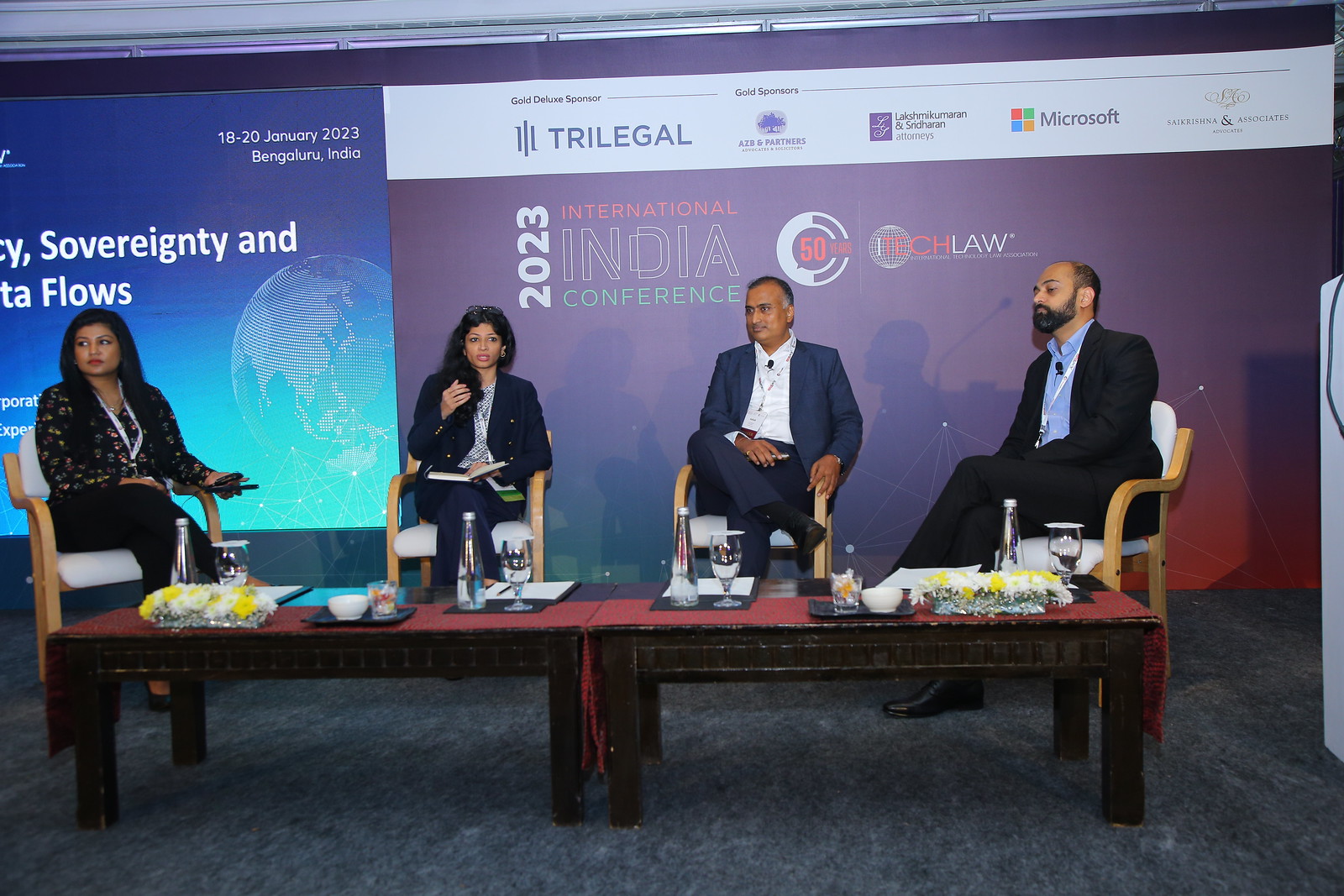This image captures a panel discussion at the 2023 International India Conference on I-Tech Law, held from January 18th to 20th in Bangalore, India. Four individuals are seated in a row of white chairs with light brown wooden accents, positioned centrally and horizontally in the frame. The backdrop prominently features a banner with the event details, including gold sponsors like Tri-Legal, AZB and Partners, and Microsoft. 

The top portion of the banner displays the text "2023 International India Conference" with complementary hues of purple, light green, blue, and touches of orange. The bottom third of the background consists of a dark gray carpet.

In front of the panelists is a low table covered with a red tablecloth, adorned with blue and brown elements and decorated with yellow flowers on each end. The table holds bottles of water, cups, and bowls of what appears to be food. 

The attendees are formally dressed, three of whom are in blue and black suits, while one woman in the center is distinguishable by her outfit consisting of a brown pair of pants and a blue jacket. The setting gives the impression of a professional roundtable discussion at a prominent international tech law conference in India.